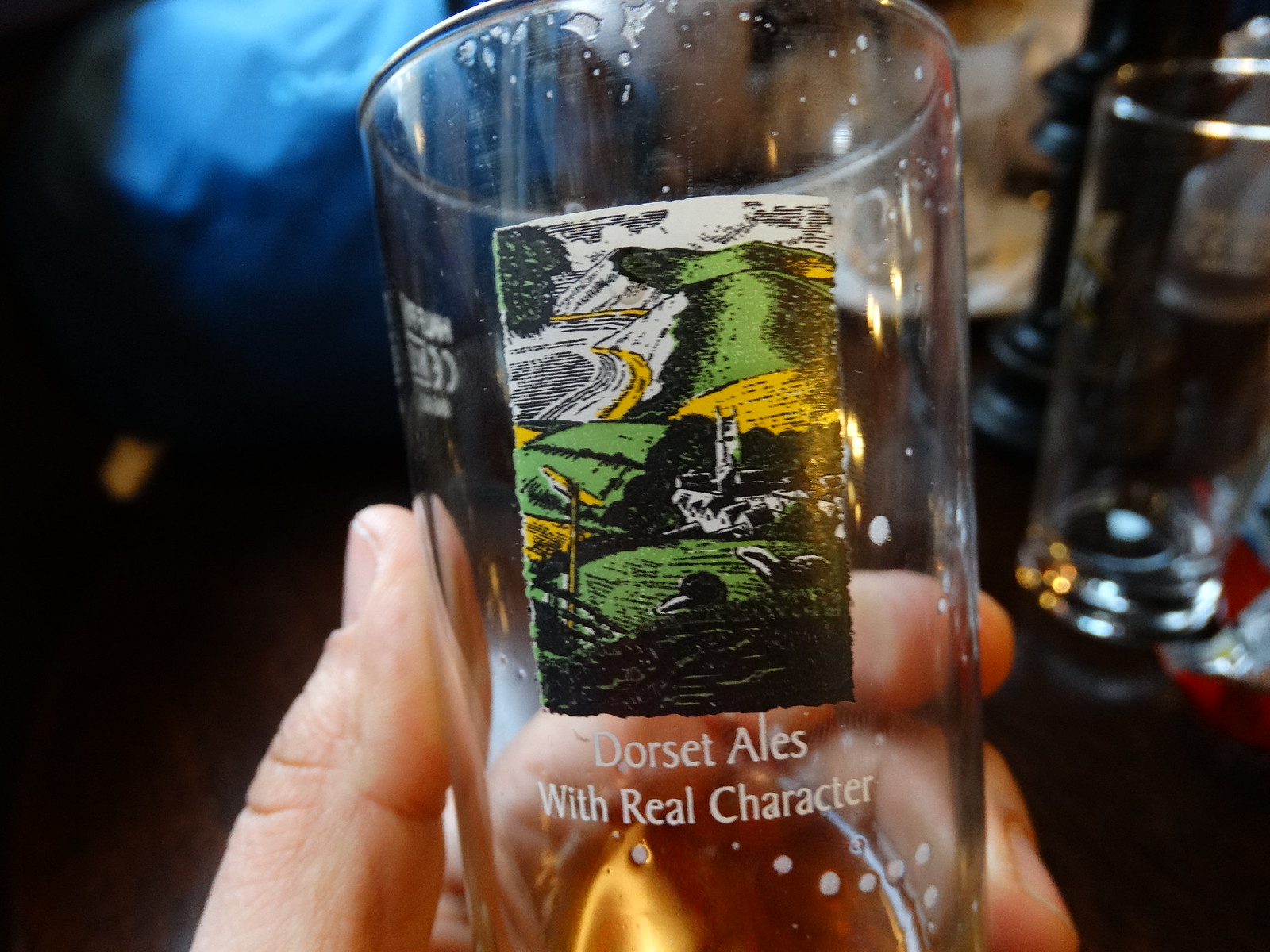In this detailed photograph, taken indoors, likely in a bar, a well-groomed Caucasian left hand is prominently featured at the center, holding a clear glass partly filled with a beverage. The glass is inscribed with a graphic depicting a green field with yellow accents and bears the text "Dawson Ales with real character." Bubbles are visible within the glass, adding texture beneath the inscription. The background is blurred, revealing an empty glass placed on a brown piece of furniture to the right and a blue jacket or towel draped over a chair to the left. The overall color palette is a mix of black, blue, yellow, brown, tan, gold, various shades of green, and red, with the bottom portion of the image showing a dark floor.